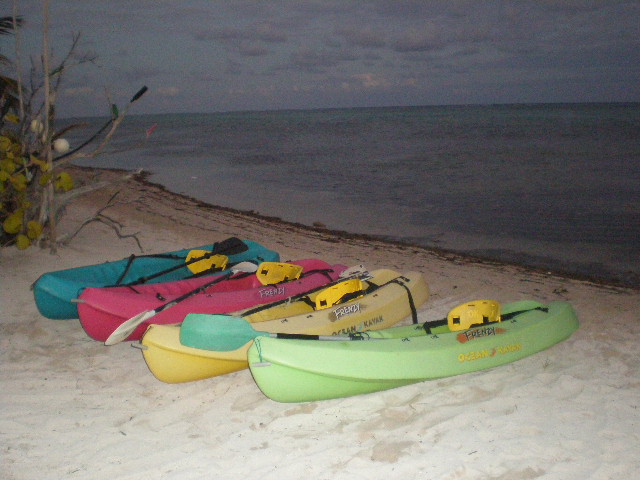In this color photograph taken at sunset, a sandy beach extends across the foreground, adorned with four kayaks aligned neatly from front to back. The closest kayak is a light green hue, featuring a matching green paddle and a yellow seat marked with "Ocean Kayak Frenzy." Next is a vibrant yellow kayak, also with a corresponding yellow paddle and seat. The third kayak is red with a lighter red paddle, while the furthest kayak is an aquamarine blue, accompanied by a black paddle. The ocean in the background deepens in shade from dark turquoise to lighter tones, contrasted against a dusky sky where clouds drift above the horizon. On the left side of the image, patches of plant life and dead wood add a touch of wilderness to the serene setting. The sky is variegated with different shades of blue and hints of light turquoise, capturing the tranquil transition from day to night.